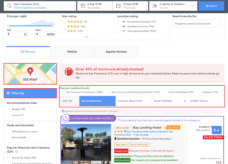This image captures a webpage interface displayed on a computer screen. At the top of the page, a black banner spans the width of the screen, featuring three white rectangles followed by a blue rectangle with white text. Scrolling down, the page showcases different rating sections, each denoted by a varying number of stars, starting with five stars at the top, followed by four, and then three stars. A prominent blue line is drawn in the upper left corner, extending slightly into a tab at the bottom.

On the left side of the page, there's a map area, highlighted with a blue rectangle bordered in red, emphasizing the location. Further down, in the middle section, a white rectangle is accented with red markings, drawing attention to that particular portion of the page. The bottom of the webpage displays a picturesque scene featuring palm trees set against a stunning blue sky, with charming houses in the background.